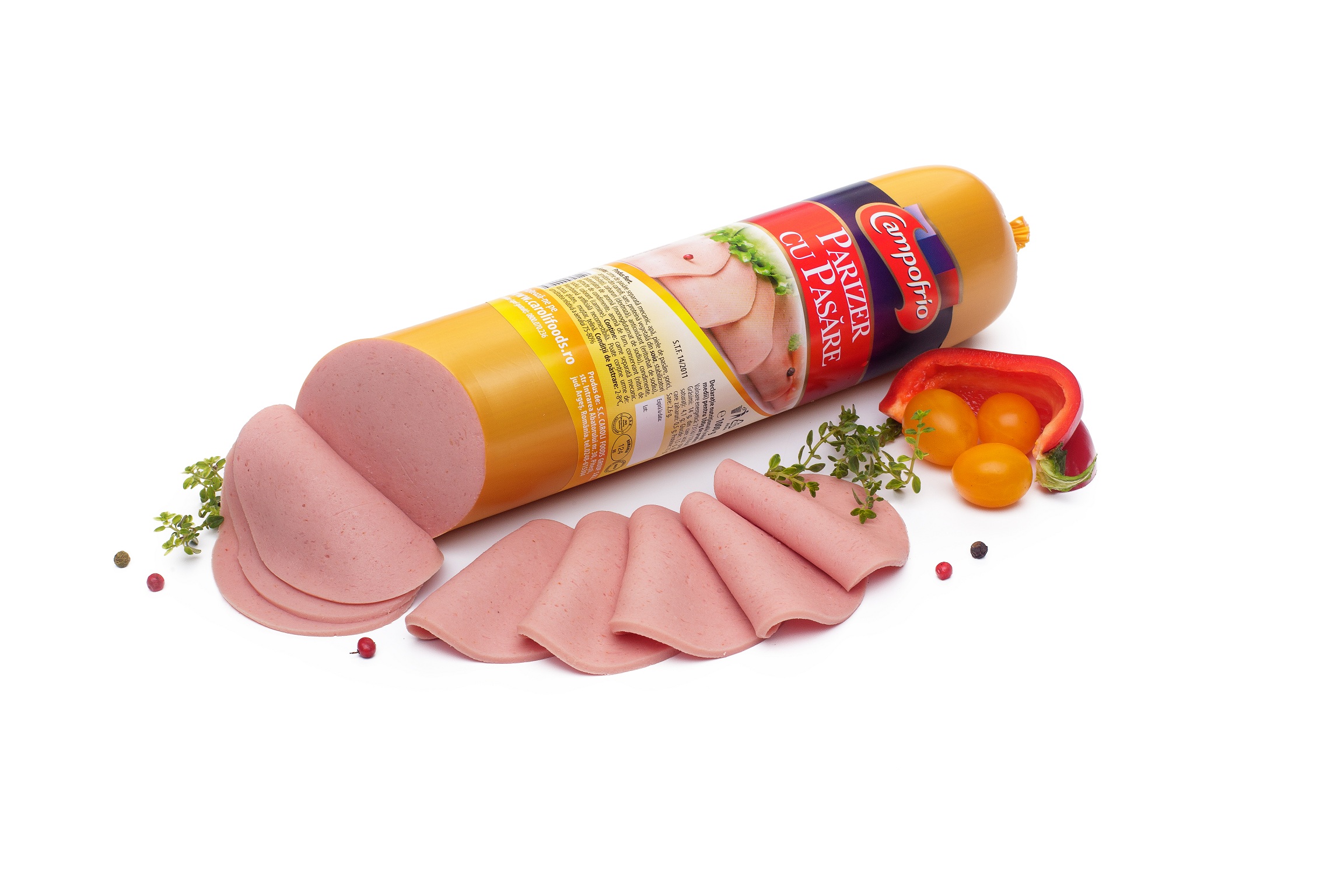On a white background, the image features a large cylindrical tube of bologna, wrapped in a predominantly yellow label with various details, such as the brand "Campo Frio Pariser" displayed prominently. This deli meat, light red in color, has been partially sliced at one end, with the slices neatly folded in front of the intact portion. Surrounding the bologna, there are assorted garnishes including green leaves, herbs, capers, peppercorns scattered throughout, three yellow cherry tomatoes, a cut red tomato, and a slice of red bell pepper in the upper right corner. The label on the bologna includes foreign text, likely in French, and features a photo of the bologna itself with decorative red, blue, and orange bands. Lastly, detailed fine print can be seen near the bottom of the label beneath the image of the bologna.